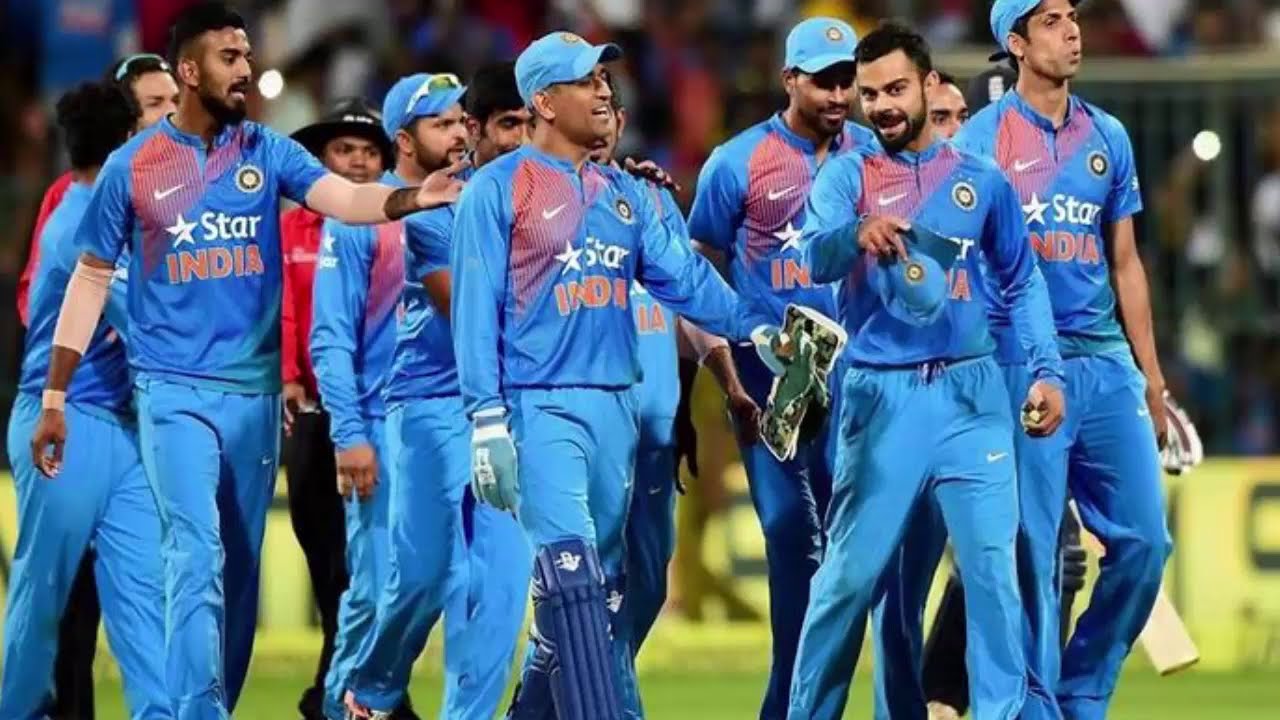The image depicts a cricket team, centrally positioned on a grassy field at an outdoor sports stadium during the day. The team consists of around ten men, all wearing blue uniforms emblazoned with 'Star India' and a five-pointed white star. The uniforms feature additional details such as the Nike logo on the right shoulder. The word 'India' is prominently displayed in red with white pinstriping. Notably, one player at the front is equipped with shin guards or knee pads, a glove on his right hand, and holds an item in his left arm. This player's companions include another individual with peach-colored sleeves and a matching wristband. Four members of the team wear blue baseball caps. The men have dark hair and medium to darker toned skin. The backdrop includes a blurred audience, advertisements, and various signs, adding to the vibrant and bustling atmosphere of the stadium.